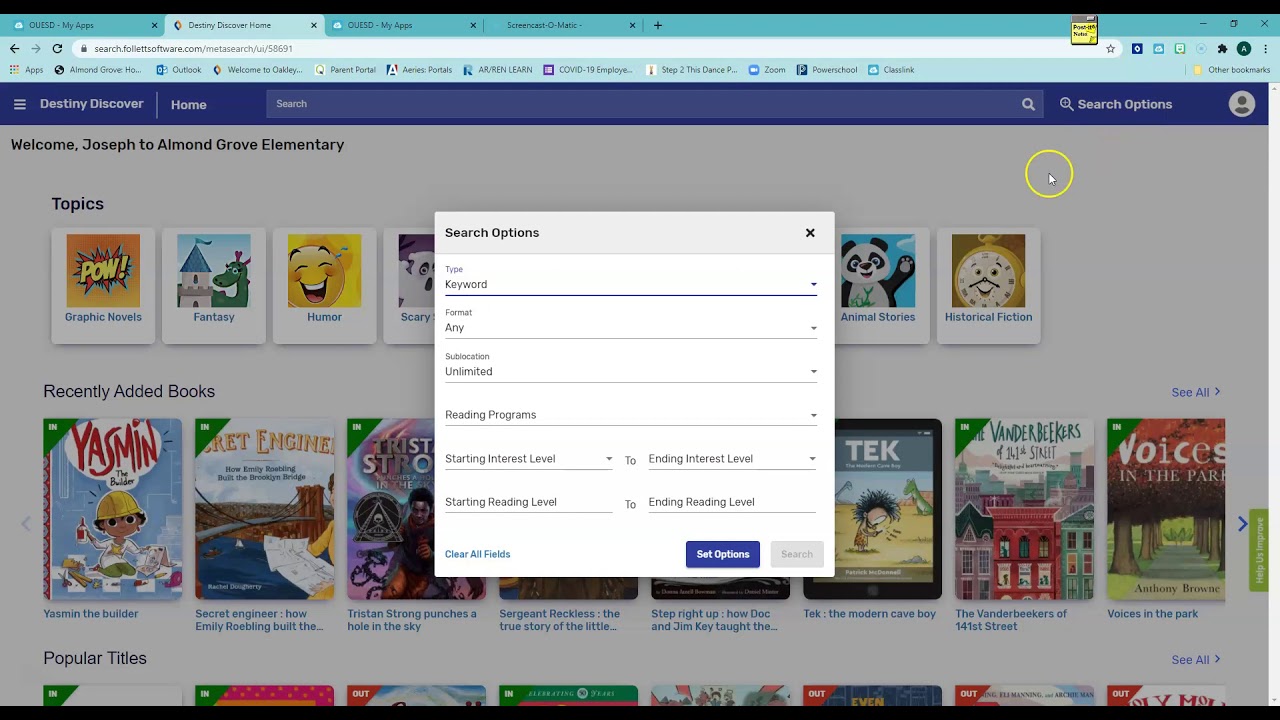The image depicts a cluttered website interface with multiple elements displayed on a computer screen. The webpage features four tabs at the top, although the small size makes them difficult to read. Below the tabs is a search bar. At the bottom of the screen, there is an address bar and a variety of bookmarks nearly filling up the bookmark space.

The main content of the webpage centers around the "Destiny Discover" platform, displayed prominently on a purple navigation bar. The bar includes options such as "Destiny Discover," "Home," an empty search bar, and account settings represented by a default avatar icon. The background of the site is white, and on the top left corner, there is a welcome message that reads, "Welcome Joseph to Almond Grove Elementary."

Various children's book covers are scattered across the page. However, the central focus is a pop-up window for search options. This window has multiple drop-down menus labeled as follows: Type (Keyword), Format (Any), Subscription (Unlimited), Reading Programs, Starting Interest Level, Starting Reading Level, Ending Interest Level, and Ending Reading Level. This pop-up box dominates the center of the webpage, making the rest of the site appear blurred in the background.